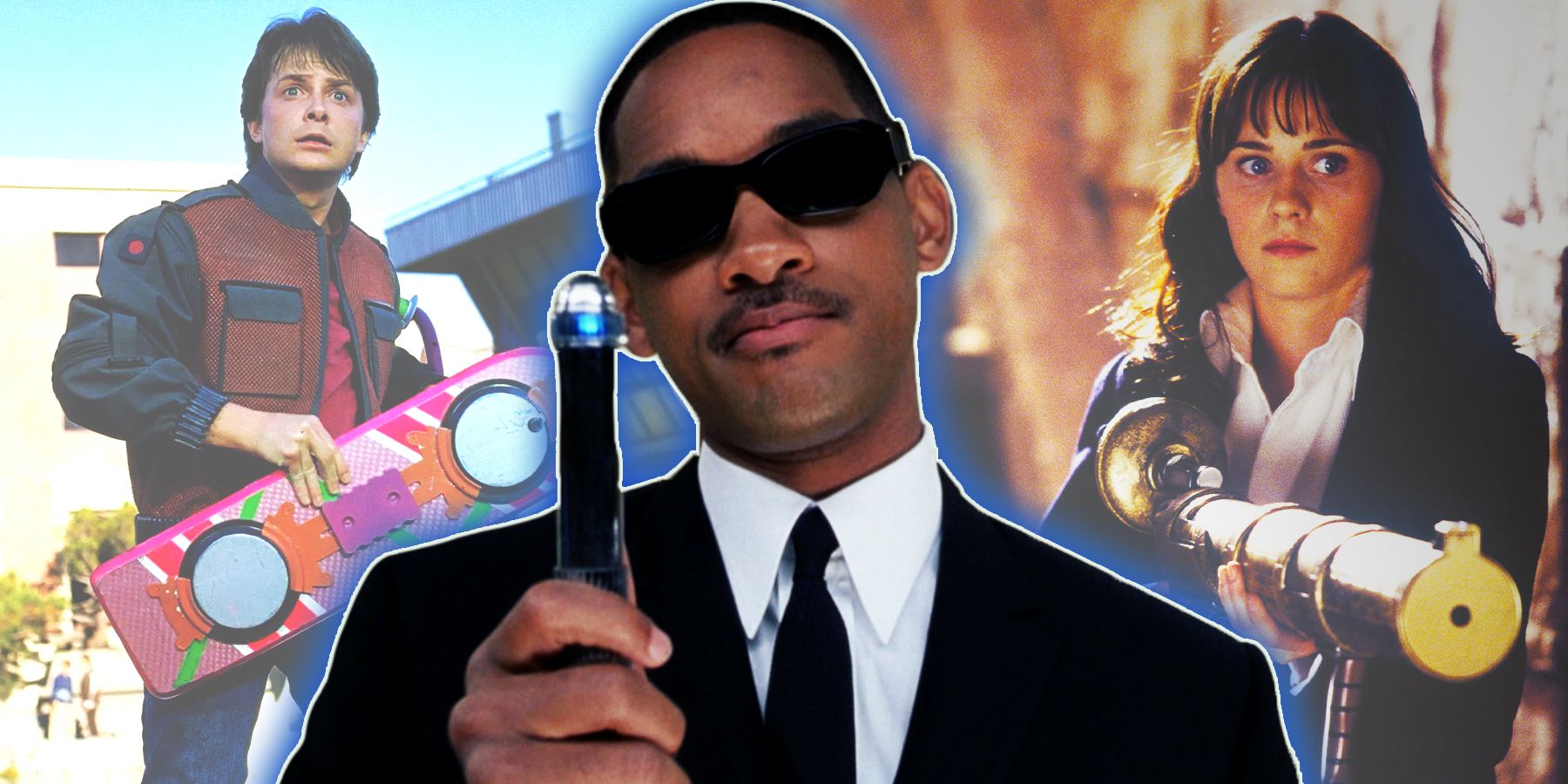In this composite image blending iconic characters from well-known movies, Will Smith from "Men in Black" stands in the center, immediately catching the viewer's attention. He dons black sunglasses and a sleek black and white suit. In his hand, he clutches the Neuralyzer, a device used to erase memories. To his left, in the background, is Marty McFly, played by Michael J. Fox in "Back to the Future." Marty sports his signature red and blue jacket and grips his pink and blue hoverboard, recognizable by its two round circles. He appears to be looking towards something intriguing off-camera. On the right side, also in the background, a woman with long brown hair and bangs commands attention. She wears a white collared shirt under a blazer and holds a large, futuristic-looking gun, aimed and ready. The image seamlessly integrates these three characters, merging their distinct cinematic worlds into a single, captivating scene.